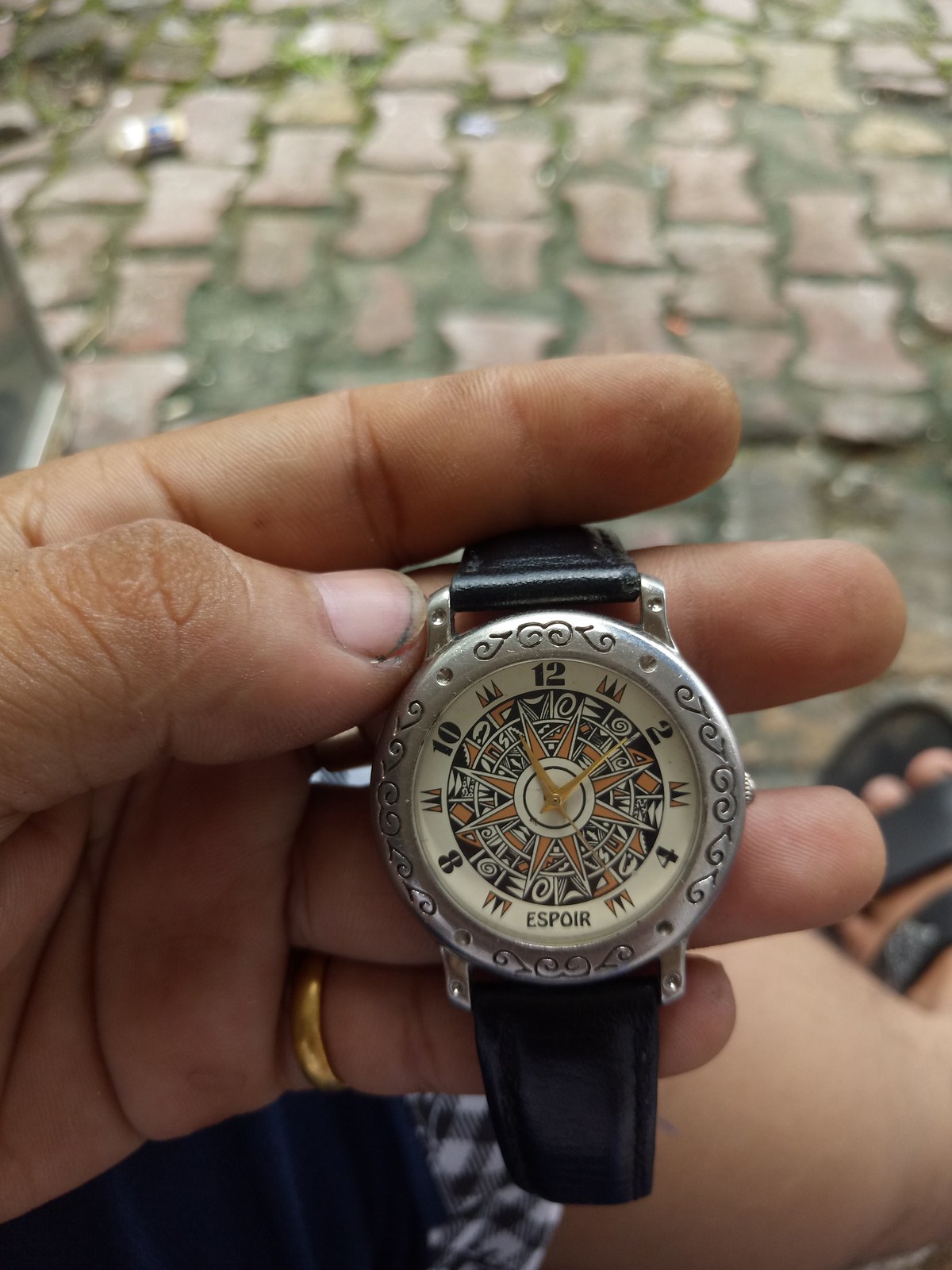This detailed color photograph features a close-up of a person's left hand holding a decorative wristwatch. The watch, secured by a black leather band, showcases a distinctive silver bezel adorned with intricate engravings. Its face is a vibrant sunburst design, accentuated by an array of browns and yellows, reminiscent of an Aztec motif. The numerals 12, 2, 4, 8, and 10 are prominently displayed, while the position of the 6 is occupied by the word "ESPOIR." The watch hands appear to be a slightly tarnished yellow. Notably, the individual wearing the watch has a gold ring on their pinky and dirt under their nails. The background reveals a blurred outdoor setting with worn stone or brick tiles, and partially visible is a foot in sport sandals, adding a rustic touch to the scene. The overall focus remains sharply on the intricate details of the watch and the hand holding it.